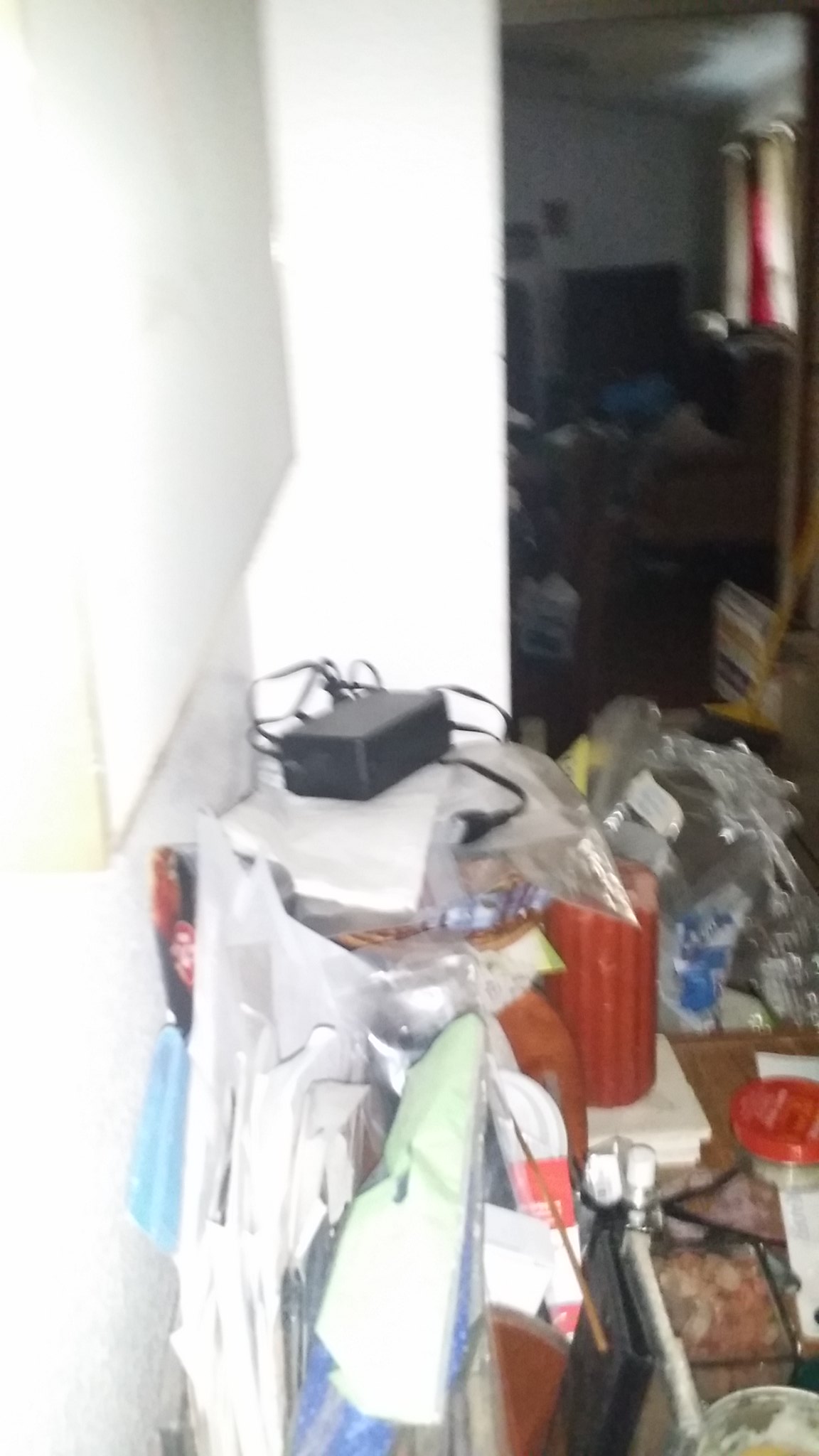This photo, although slightly blurry and dimly lit, captures the cluttered interior of a home. The foreground features a room with white walls and a dirty, pinkish-hued tile floor, barely visible beneath the myriad of items scattered across it. The room is overwhelmed with piles of plastic bags, stacks of papers, and an array of miscellaneous objects, creating an impression of a hoarder’s living space. In the background, another room can be seen, equally dark and cluttered, with closed or partially closed curtains on the window. This room also holds numerous boxes and plastic bottles strewn across the floor, contributing to the overwhelming sense of disarray in the home.